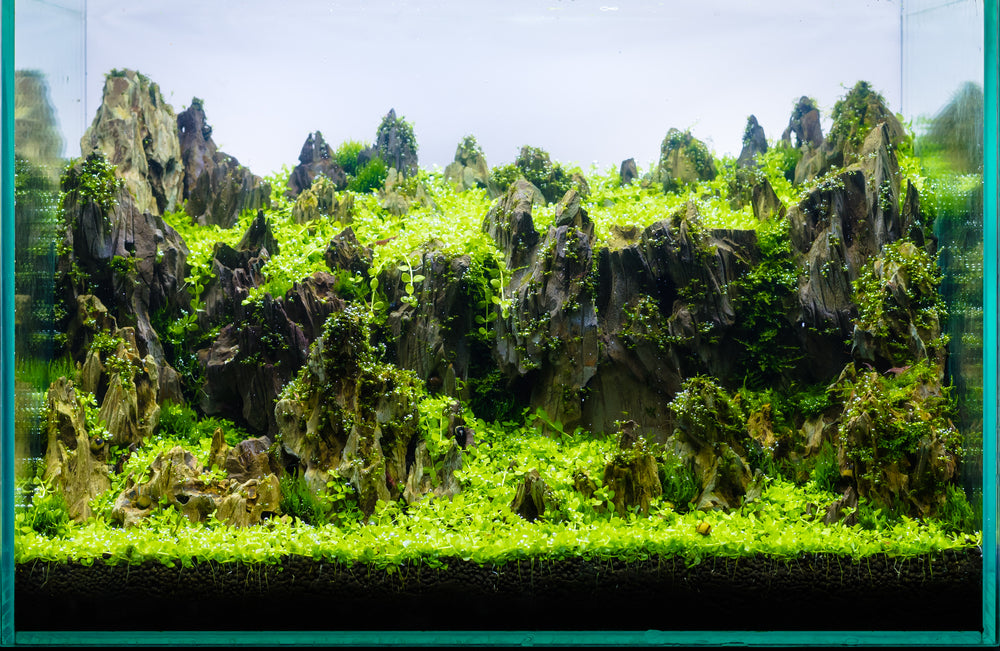The image depicts a detailed and vibrant photograph of the inside of a terrarium or reptile enclosure, characterized by its glass sides and back, hinting at an enclosed tank environment. Inside the tank, the layered, jagged brown and gray rocks dominate the scene, their surfaces densely covered with light green, delicate foliage and thick moss. Several vine-style plants cascade down the rocks, adding to the lush, verdant atmosphere. The dense vegetation, featuring many small and fragile leaves, completely envelops the rocky terrain, creating a rich, green tapestry. A hint of condensation is visible on the glass walls, enhancing the sense of an enclosed, humid ecosystem. In the background, there is a bluish tint, possibly an image meant to simulate the sky, contributing to the illusion of an outdoor landscape within this miniature, meticulously crafted display.